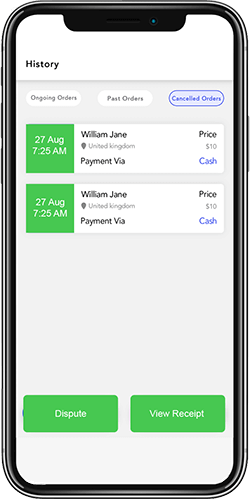The image depicts a highly realistic drawing of a smartphone, showcasing both the screen and the phone’s frame in shades of gray and silver. The screen displays a detailed interface with a white header at the very top, where "History" is written in black font on the left side. Below this header, the background shifts to a very light gray.

In this section, there are three white, rounded rectangles aligned horizontally. The first rectangle has "Ongoing Orders" written in grey font, the middle one reads "Past Orders," and the third rectangle is bordered by a blue line with "Canceled Orders" written in blue font.

Further down, the screen showcases two additional white rectangles, each containing detailed information. The first rectangle displays "William Jane" on the left. To the right, it reads "Price," followed by "$10" underneath. Adjacent to this price tag is a slightly wider green rectangle with the text "27 AUG 7:25 AM" written in white font. A similar white rectangle appears below, repeating the details: "William Jane," "Price," "$10," and "Cash," with a green rectangle to the left that also says "27 AUG 7:25 AM" in white font.

At the very bottom of this screen, two green rectangles are highlighted. The one on the left reads "Dispute" in white font, while the right one says "View Receipt" also in white font.

This image effectively portrays a well-organized and detailed interface for managing orders on a smartphone.